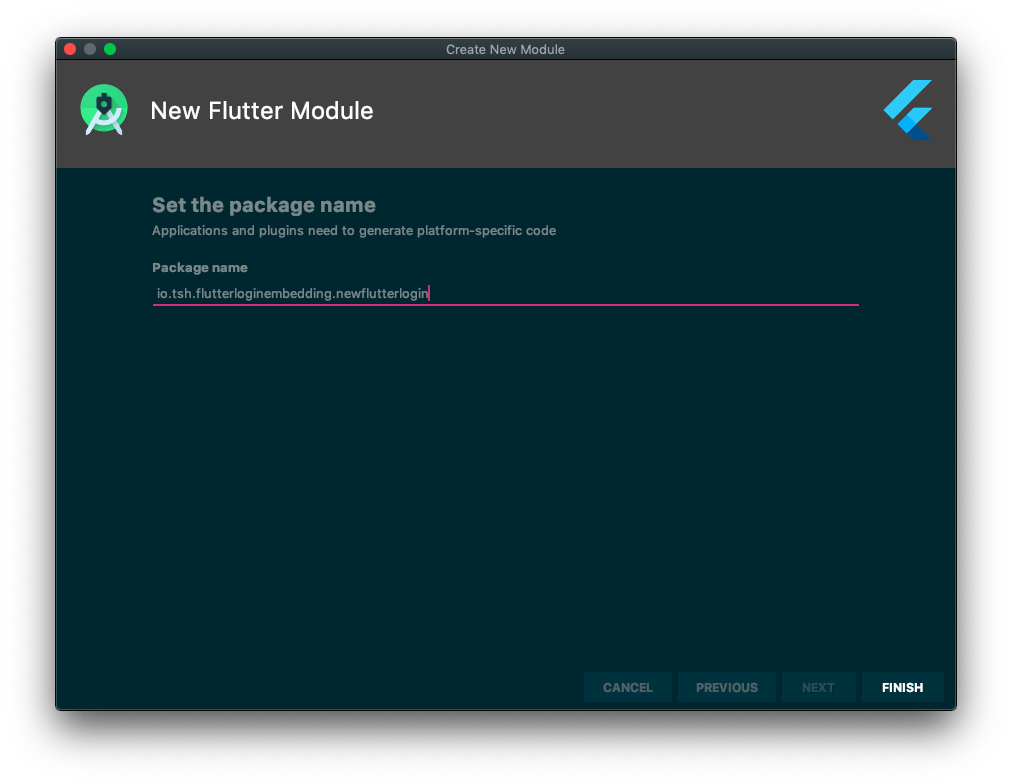The image is a screenshot of a user interface, presumably from a software development environment. At the very top of the screen, there is a black bar featuring three dots on the left side: an orange dot, a grey dot, and a green dot, indicating typical window control buttons. In the center of this black bar, there is text that reads "Create New Module."

Below this top bar, there is a large grey box with the heading "New Flutter Module" written in prominent white text. Within this grey box, there is a green circle that contains an image icon resembling a camera on a tripod, possibly hinting at a project type or template.

Towards the right side of the grey box, there are two overlapping paper icons; one is depicted as folded while the other is flat. This might indicate document or file options.

Moving down to another black section of the interface, there is a prompt labeled "Set a Package Name." This section explains that "Applications and plugins need to generate platform-specific code." Below this instructional text, the package name is displayed as "io.tsh.flutterloginembedding.newflutterlogin." This package name is underlined in pink, with a vertical pink line cursor positioned immediately after the "N" in "newflutterlogin," suggesting that this field is currently active or being edited.

At the bottom of the screenshot, there is a navigation bar with four buttons: "Cancel," "Previous," "Next," and "Finish." The "Finish" button is highlighted, indicating that the user is likely ready to complete the process.

This detailed description gives a comprehensive overview of the visual elements and layout presented in the screenshot.